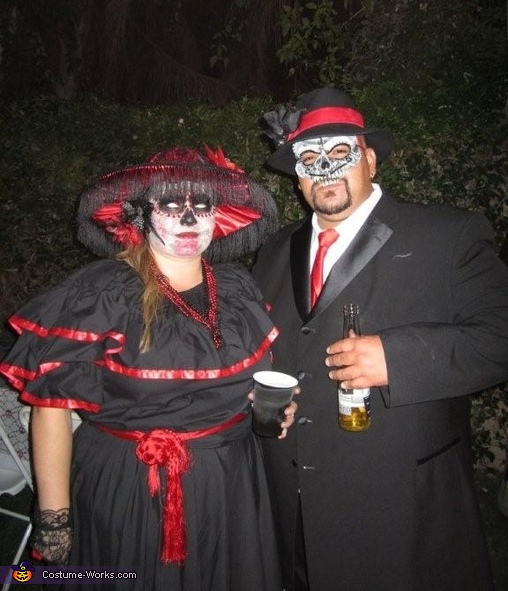The photograph captures a couple at a nighttime costume party, identified by the "CostumeWorks.com" label in the bottom left corner. The background reveals dark, leafy shrubbery illuminated by a camera flash. The couple is dressed in elaborate Halloween costumes with a strong Day of the Dead or Mardi Gras theme.

The man stands on the right, wearing a black tuxedo, white dress shirt, and a red tie. His face is adorned with skull-like face paint, highlighting his eyes, nose, cheekbones, and teeth. He sports a black gangster-style hat with a red band and a black rose on the side. In his left hand, he holds a Corona beer bottle.

The woman, positioned on the left, is dressed in a black ruffled dress accented with a red belt and red trims. Her face is completely covered in intricate skull face paint, and she wears a dramatic black hat with red tassel fringe, possibly inspired by Mexican or Hispanic designs. She accessorizes with black gloves—one of which is lace—and her fingernails are painted black. In her hand, she holds a black solo cup.

Both individuals adopt a striking pose that emphasizes their coordinated black, red, and white attire, setting a vivid and festive tone against the dark nighttime background.